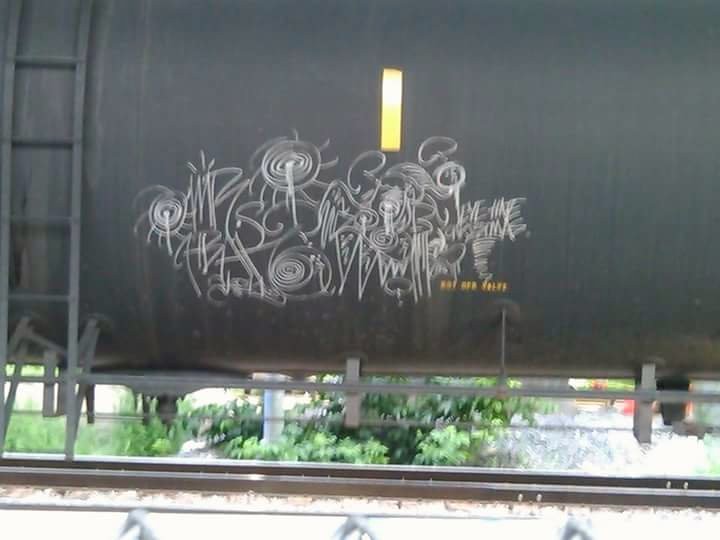The image is a blurry, close-up photograph of a dark grey train car, partially obscured, with graffiti prominently displayed on its surface. The graffiti, done in white, consists of various shapes including swirls, circles, and stylized mushrooms with wings, suggesting the work of a skilled artist. There are also blurred words that appear to be written in white chalk. On the left side of the train car, a steel ladder ascends the structure. Below the train car, partially visible train tracks and some vegetation suggest that the photograph was taken in a rail yard during the daytime. Despite the lack of focus, the image captures the intricate details of the graffiti against the industrial backdrop.